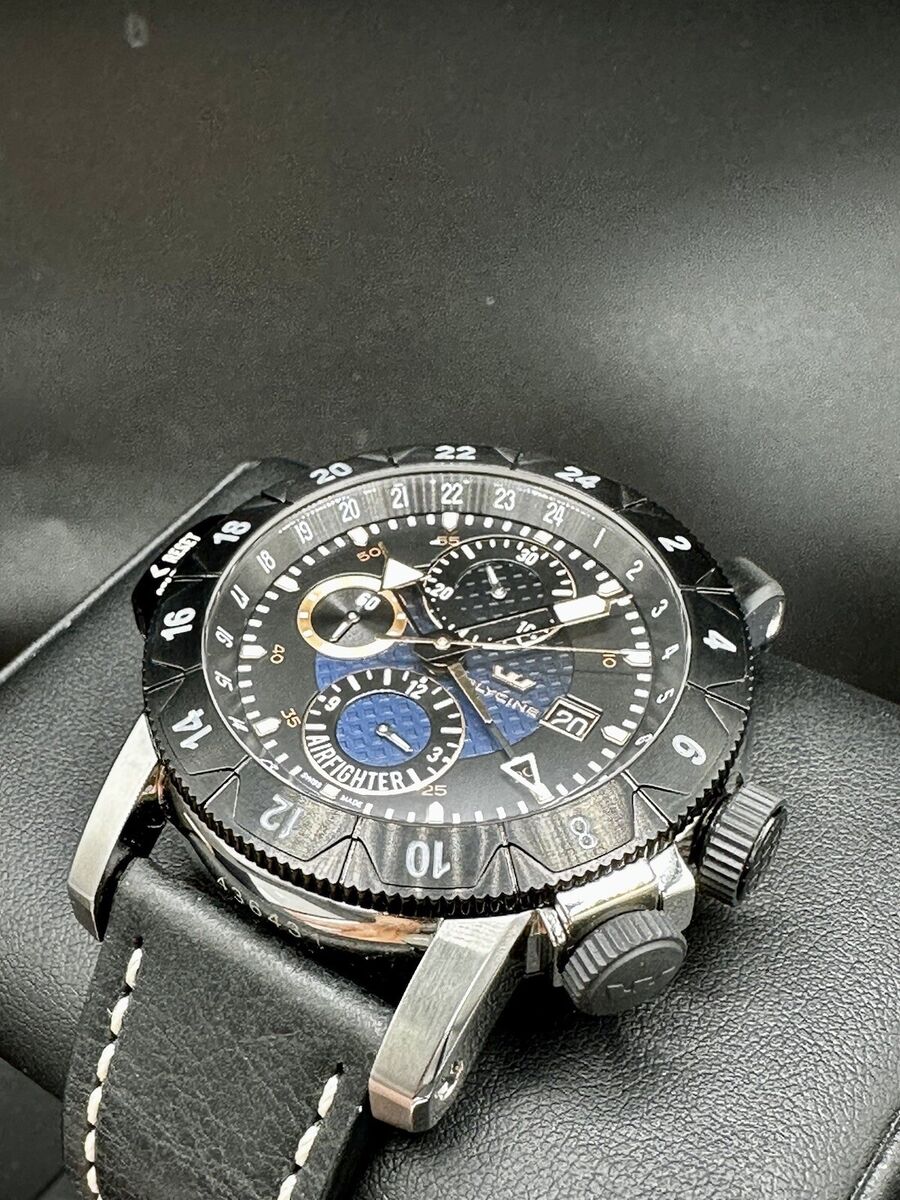In this photograph, a sophisticated men's watch is presented on a sleek black holder with a matching black background. The watch features an elegant black leather band with white stitching along its edges. The standout watch face, rendered in black and silver with intricate details, showcases multiple dials and indicators, including a standard 12-hour clock and an outer 24-hour clock, seamlessly adorned with blue, black, gold, and white accents. The face is marked with "Air Fighter," hinting at potential aviation-related functionalities. Four distinct hands can be observed: a black hour hand with a solid white arrow tip, a black and silver minute hand with a hollowed-out white triangular tip, a slender second hand, and a thicker fourth hand. The watch also includes two dials on the side for adjustments. The entire assembly is angled diagonally from right to left, positioned atop a textured black leather material, likely a folder or wallet, which adds an extra layer of sophistication to the overall presentation.